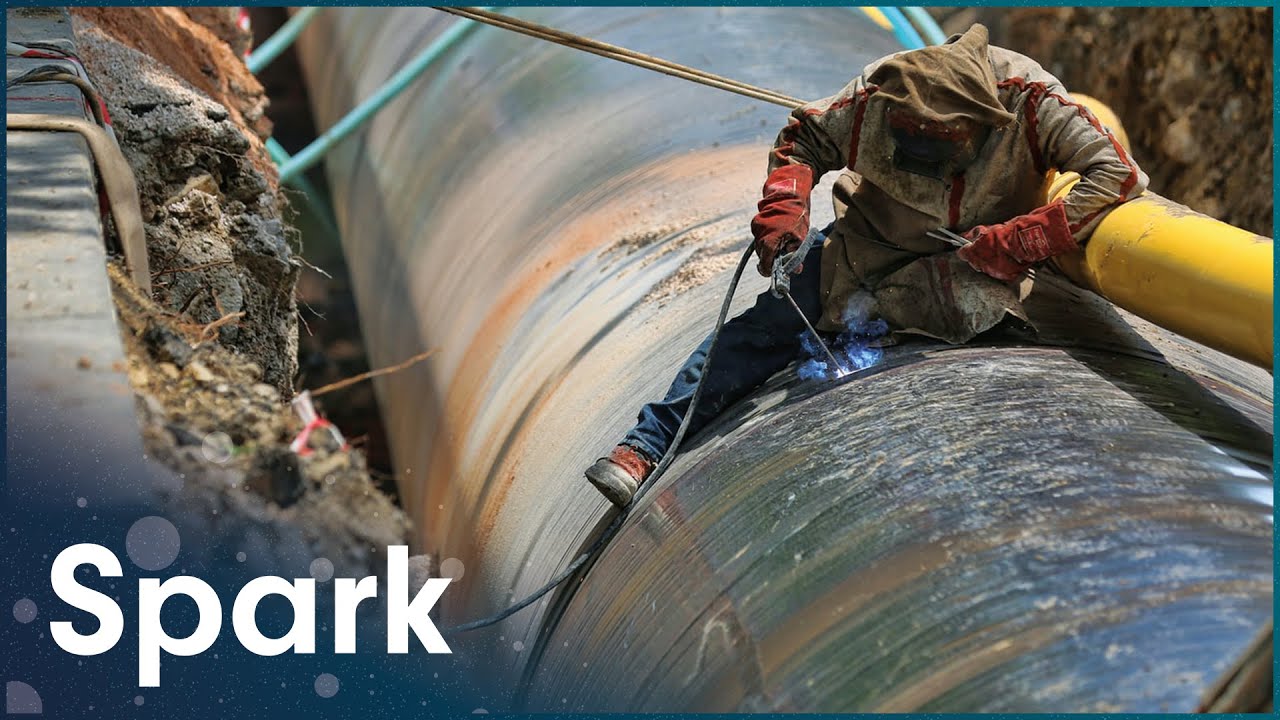The image depicts a color photograph of a man welding inside a deep excavation, lined with dirt and rocks. Central to the image is a large black pipe or tube. The man, dressed in blue jeans, work boots, red welding gloves, and a protective tan jacket with red stripes, is engaged in welding the pipe. He wears a welding mask and leans his forearm against a smaller yellow pipe, holding two metal welding rods in one hand while operating the welder with the other. Blue flames can be seen emanating from the spot where he touches the metal rod to the pipe. A rope is attached to him, trailing from the left corner of the image. The word "SPARK" is prominently displayed in white letters in the bottom left-hand corner of the photograph.